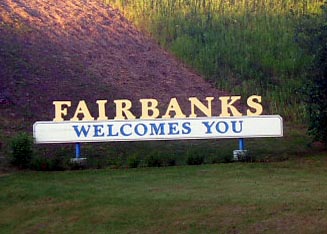This photograph captures a detailed outdoor scene featuring a welcoming sign for Fairbanks. At the base of the image, there is a field of grass displaying a mix of green and brownish-red patches. The sign itself comprises individual uppercase letters spelling "Fairbanks" in a yellowish beige hue mounted on top of a white rectangular panel. Below these letters, the words "welcomes you" are prominently displayed in blue font on the white panel. The entire sign stands on two sturdy blue poles. Surrounding the sign are patches of green grass and short shrub-like plants. In the background, to the left, there are clusters of purple lilacs, adding a touch of color to the scene. To the right, green leaves from a large bush or tree extend into the frame. The overall landscape behind the sign includes a mixture of brown dirt and long, green grassy areas, suggesting the presence of a hill or slope. The sunlight casts a warm glow across the fields and foliage, enhancing the colors and adding to the welcoming atmosphere portrayed in the image.